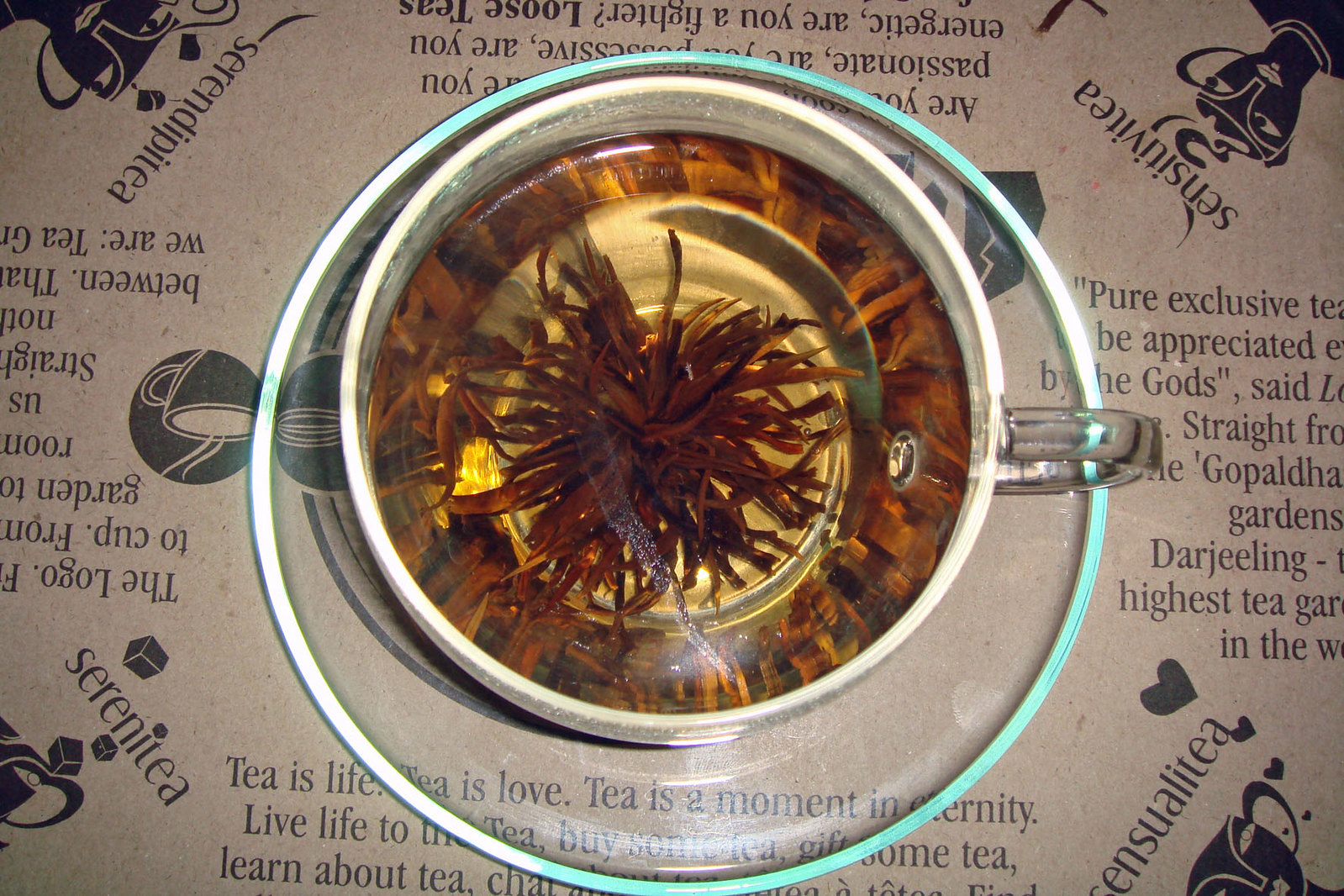This is a detailed photograph taken from above of a clear, see-through glass teacup filled to the brim with a clear liquid, likely water, and containing what appear to be dark brown or orange tea leaves arranged in a manner reminiscent of a sea anemone, with multiple spaghetti-like strands extending from a central point. The teacup is placed on a matching clear saucer, which rests on a placemat that resembles a newspaper or a cardboard design. The placemat contains various tea-related quotes, including "tea is life, tea is love, tea is a moment in eternity," partially obscured by the bottom of the image. The overall scene suggests a deep appreciation for tea, adding a touch of whimsy and intrigue with the unusual arrangement of the tea leaves.